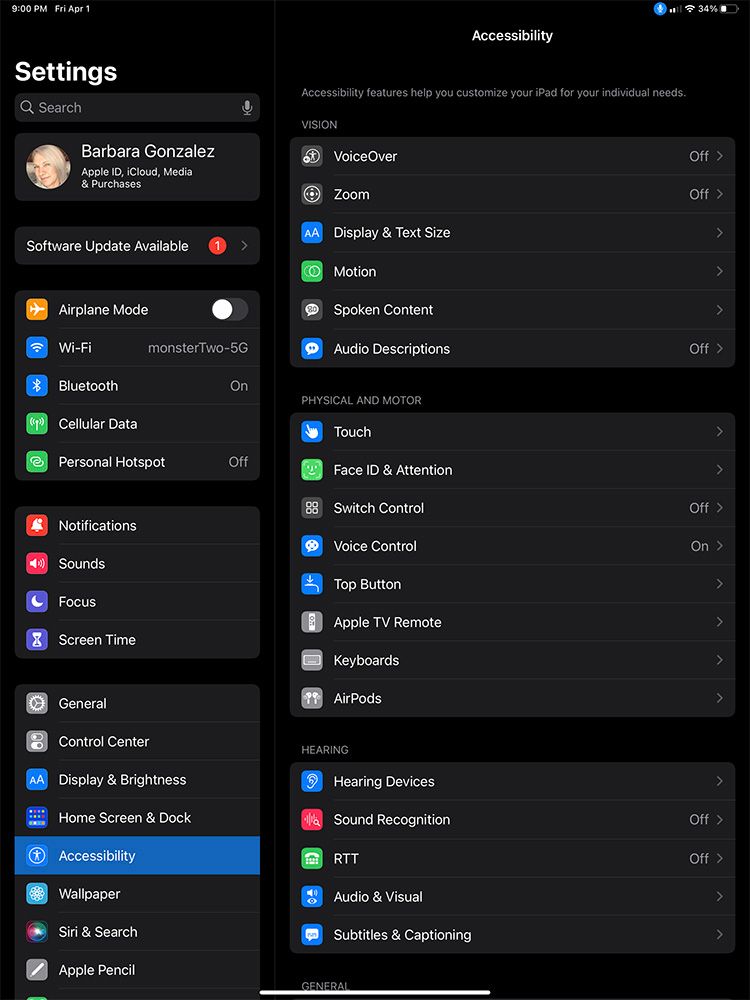This detailed screenshot showcases Barbara Gonzalez's Apple ID and various device settings. The image features a black background with a prominent blue rectangle highlighting specific options. Notably, a software update is available. Key settings include:

- **Airplane Mode**: Enabled
- **Wi-Fi**: Connected to "Monster 2" (5 GHz)
- **Bluetooth**: Enabled
- **Cellular Data**: Disabled
- **Personal Hotspot**: Disabled

Other menu options listed are:
- Notifications
- Sounds
- Focus
- Screen Time
- General
- Control Center
- Display & Brightness
- Home Screen & Dock
- Accessibility (expanded with sub-options shown)

Among the Accessibility options, notable settings are:
- VoiceOver
- Zoom
- Display & Text Size
- Motion
- Spoken Content
- Auto-Descriptions: Off
- Physical and Motor abilities:
  - Touch
  - Face ID & Attention
  - Switch Control: Off
  - Voice Control: On
  - Top Button
  
Additionally, device controls and integrations include:
- Apple TV Remote
- Keyboards
- AirPods
- Hearing Devices
- Sound Recognition: Off
- RTT (Real-Time Text): Off
- Audio/Visual options
- Subtitles & Captioning

In summary, this screenshot encapsulates Barbara Gonzalez's Apple ID and diverse settings, illustrating her device preferences and configuration.